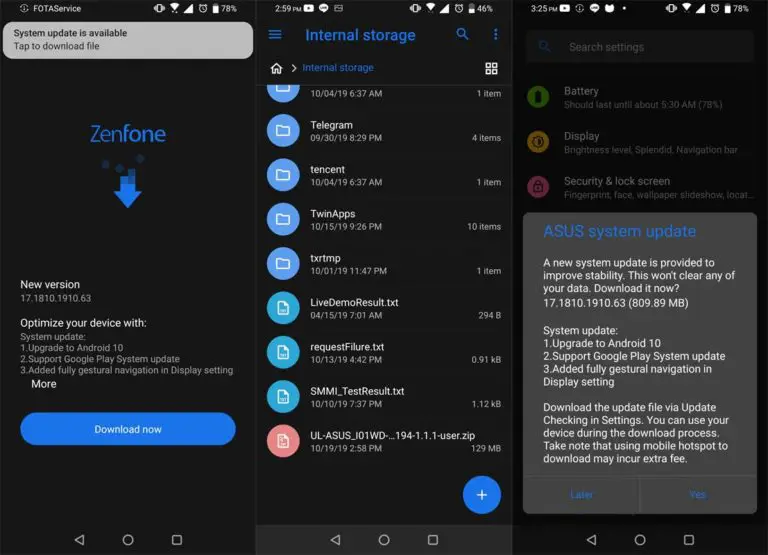Here is a detailed and cleaned-up caption for the image described:

---

The image comprises three separate screenshots from a mobile device, formatted vertically. 

1. **Left Screenshot:**
   - The top of the screen shows the "Photoservice" application with a charcoal gray or black background.
   - A notification bubble states, "System Update is Available. Tap to download file."
   - Below the notification, the "Zenfone" logo appears in blue, characterized by three additional blue dots and a downward-pointing blue arrow.
   - Different sections follow, headed by "New Version," offering device optimization details and a blue button labeled "Download Now" in white text.
   - At the bottom are typical navigation buttons for the device: Home, Back, and a Square button.

2. **Center Screenshot:**
   - The top header reads "Internal Storage" in blue text against a charcoal black background.
   - Listed below are various files and folders typical of phone storage, such as "Telegram," "Tencent," and "Twin Apps."
   - Specific text files are named "Live Demo Result.TXT" and "Request Failure.TXT."
   - File icons include a plain file symbol resembling a vanilla envelope with a light blue background, and a plain text file silhouette over a light green background.

3. **Right Screenshot:**
   - Features a notification window with a light gray background against a charcoal black backdrop.
   - Titled "ASUS System Update" in blue text, the notification message reads: “A new system update is provided to improve stability. This won’t clear any of your data. Download it now.”
   - Details of the update include "System Update 1," enumerating:
     1. Upgrade to Android 10
     2. Support for Google Play System Update
     3. Added fully gestural navigation and display settings
   - Instructions follow, advising to download the update file via settings, noting possible fees for using mobile hotspots.
   - At the bottom, two options appear: "Later" and "Yes," both in blue text.

---